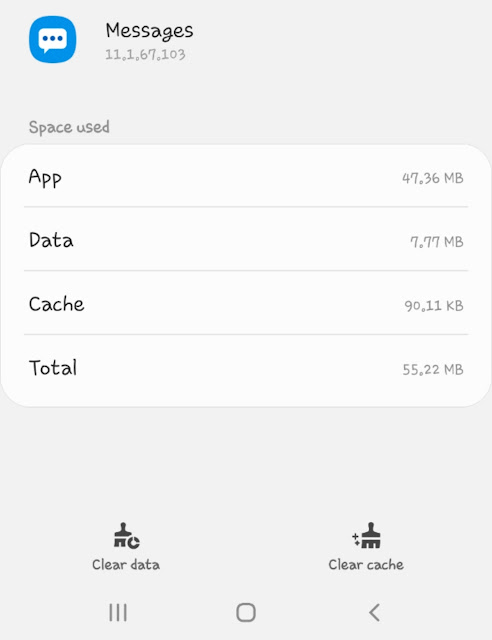The image depicts a webpage with a gray background that appears to be related to data and app storage management. At the top, the page is titled "Messages." A blue circle containing a white square with four dots arranged in a cross pattern is prominently displayed. Below the title "Messages," it shows the version number "11.1.67.103."

The webpage provides detailed information on the storage space used:
1. App: 47.36 MB
2. Data: 7.77 MB
3. Cache: 90.11 KB
4. Total: 55.22 MB

Users are given options to clear their data and cache to free up space. Under the "Clear Data" button, three vertical lines suggest the presence of a menu. In the middle of the page, there is an arrow pointing to the left, though it is not immediately clear what this arrow is associated with. The storage details indicate that the total storage space used is 55.22 MB, with an implicit suggestion that users can clear data or cache to manage or reduce this storage.

There is no indication of whether this webpage pertains to a specific device, such as a phone or tablet.